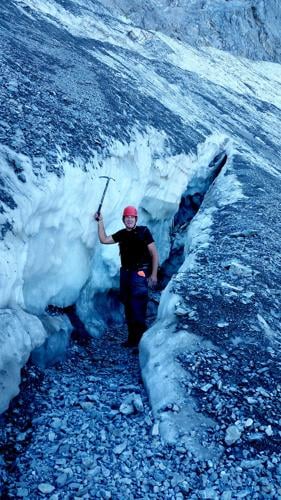The photograph captures a man standing outdoors in the mountains on an overcast day, posing with a smile despite the cold. He wears a short-sleeved black shirt, blue jeans, and a red hard hat, and he holds an ice pick aloft in one hand, suggesting a sense of achievement or perhaps involvement in a scientific endeavor. The man is positioned within a narrow crevice in a rocky mountain slope, surrounded by snow and ice, emphasizing the harsh, chilly environment. The crevice extends up the mountain wall, which is composed of solid white rock interspersed with icy patches, lending a stark, wintry backdrop to the scene. The man’s attire, unusual for the cold conditions, accentuates the ruggedness and thrill of the moment.